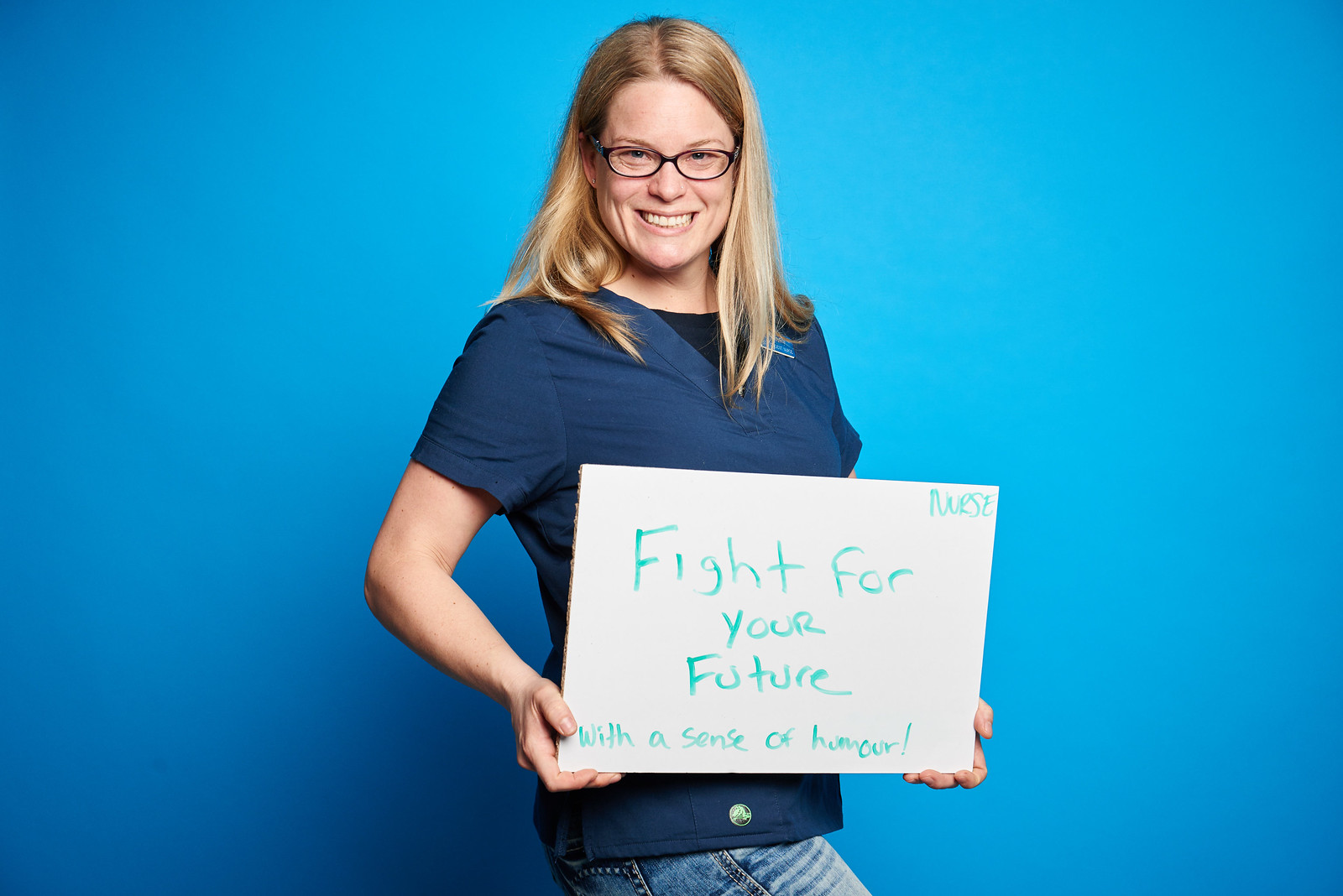The image captures a smiling woman standing against a gradient blue background, which is lighter in the center and darkens towards the edges. She appears to be Caucasian and is wearing black-framed glasses. Her blonde hair, parted in the middle, cascades down past her shoulders. She is dressed in a navy v-neck scrub top, possibly indicating a medical profession, with a darker blue undershirt visible beneath it, and light distressed wash jeans. The woman holds a bright white sign in both hands which reads in teal handwriting, "Fight for your future with a sense of humor." In the upper right corner of the sign, the word "nurse" is written, hinting at her occupation. She stands slightly angled but leans towards the camera, emphasizing her warm and engaging smile.